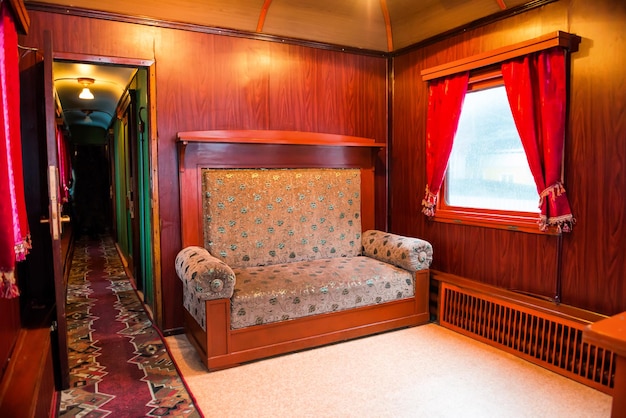This photograph depicts a cozy, small room characterized by its rich wooden elements and soft, inviting furnishings. The lower portion of the walls is adorned with reddish-brown wood paneling topped by a dark wood strip, while the upper section transitions to a pale, almost cream-colored wood. Central to the room's decor is a love seat with a sturdy wooden frame, featuring light wood at its base and a darker, reddish wood trim around the top. A darker wood strip spans the top of the back cushion, which is pale gray and made of a soft, reflective material adorned with delicate, shiny blossoms. The bolstered arms add comfort and style, with the love seat placed snugly against one wall.

Adjacent to this setup, the perpendicular wall hosts a window framed in a dark honey brown wood. The window is dressed with short red curtains, neatly pulled back with white sashes trimmed with fringe. The room's flooring includes a cream-colored area rug, beneath which lies cream carpeting. A radiator runs along the bottom of one wall, providing warmth and completing the room's snug ambience.

Leading out from this room, a door opens to a long, narrow hallway adorned with a runner rug. The rug is a striking red wine color, featuring an intricate pattern in white, black, tan, and brown, guiding the way down the passage.